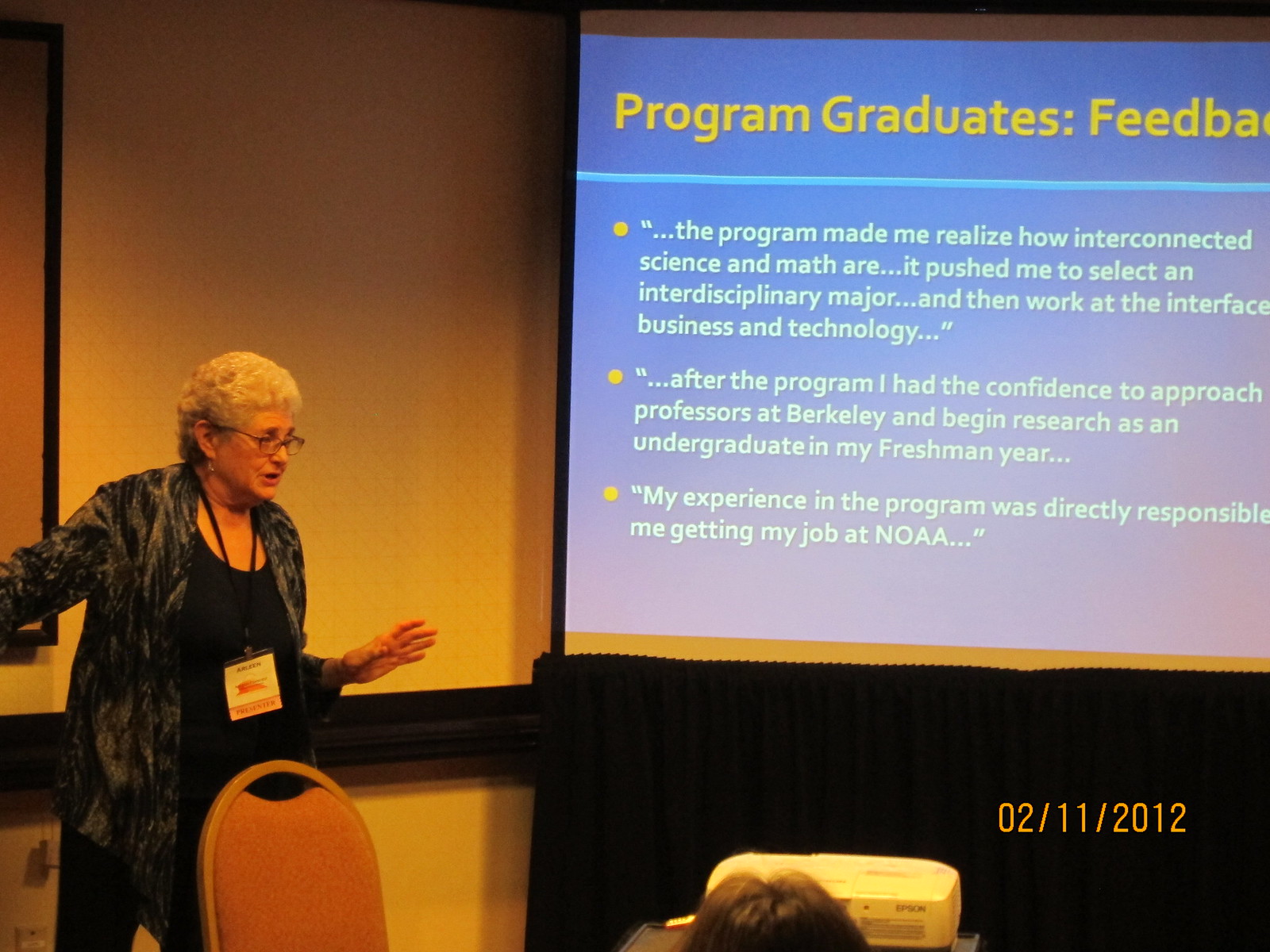An older woman with short gray hair, wearing glasses and expressive earrings, stands in a classroom-like conference room. She is dressed in a gray and black printed open sweater over a black shirt and black pants. She has a lanyard with an ID around her neck. The woman appears to be speaking to an audience, gesturing expressively with her hands. The audience isn't fully visible, but the head of one person with brown hair and an empty red-upholstered chair can be seen.

To her left, a small white Epson projector displays a presentation on a projection screen. The screen, with a blue background and yellow text, has the title "Program Graduates' Feedback." The content on the screen includes three bullet points:

1. "The program made me realize how interconnected science and math are. It pushed me to select an interdisciplinary major and then work at the interface of business and technology."
2. "After the program, I had the confidence to approach professors at Berkeley and begin research as an undergraduate in my freshman year."
3. "My experience in the program was directly responsible for me getting my job at NOAA."

The screen's projected text is organized in a sans-serif font and presented in white. A timestamp on the bottom right of the photo reads "02-11-2012."